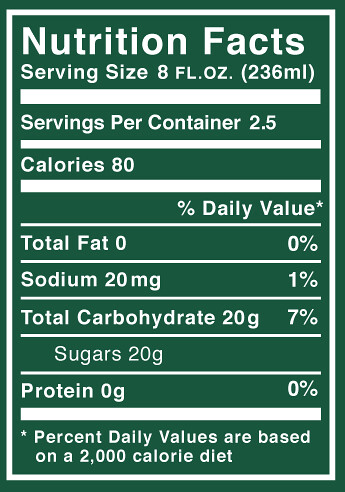The image displays a vertically-oriented rectangular Nutrition Facts label with a dark hunter green background, bordered by a white frame. The label features white, block-letter text and is divided by horizontal white bars. At the top, it reads "Nutrition Facts." Below that, it specifies a serving size of 8 fluid ounces (236 milliliters) and indicates there are 2.5 servings per container. The label details that each serving contains 80 calories, 0 grams of total fat (0% daily value), 20 milligrams of sodium (1% daily value), 20 grams of total carbohydrates (7% daily value), including 20 grams of sugars, and 0 grams of protein (0% daily value). An asterisk notes that the percent daily values are based on a 2,000 calorie diet.